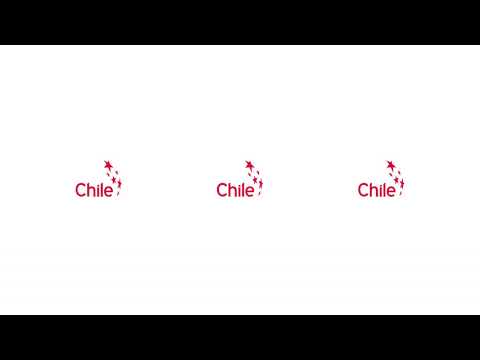The image features a clean, minimalist design with a white background and is framed by thick black borders at the top and bottom. Positioned evenly across the width of the image are three identical logos. Each logo consists of the word "Chile," stylized with a capital 'C' and lowercase 'hile' in a red font. To the immediate right of the text, there are six red stars arranged in two rows: the top row has three larger stars, and just below it, three smaller stars. This pattern of text and stars is repeated in the center and to the right of the image, creating a balanced and aesthetically pleasing composition. The overall design is simple yet effective, highlighting the word "Chile" and its associated stars against the stark white background, accented by the parallel black borders at the top and bottom.